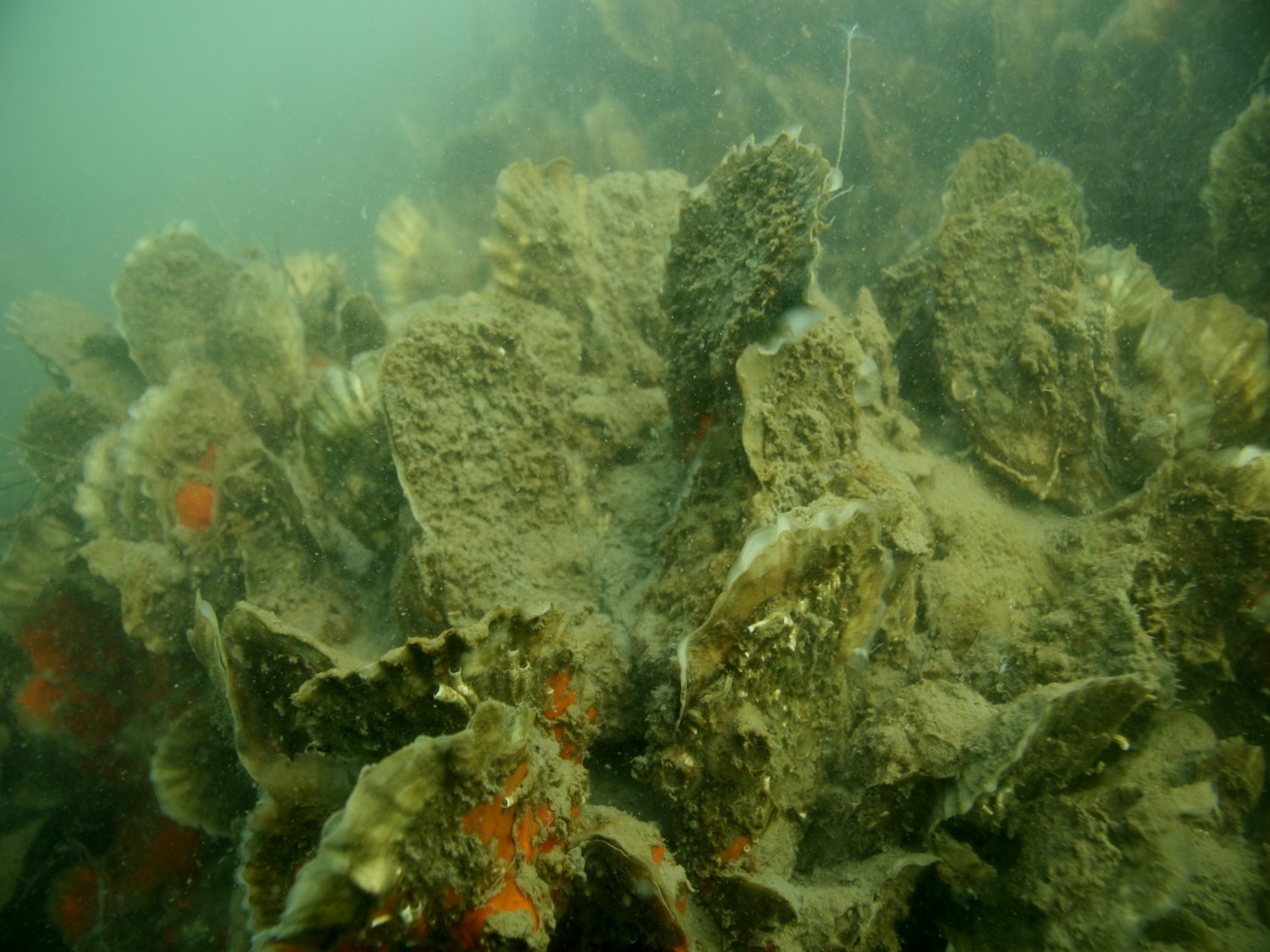This underwater photograph captures a view of a murky coral reef, enveloped in shades of green and grayish-green hues, suggesting a cloudy and somewhat dirty environment. Central to the composition is a prominent chunk of rocky, leaf-like coral, predominantly dark green with reddish-orange hues accentuating its rough, petal-like appendages. The front of the image features this striking coral piece, while the background reveals additional, slightly blurred coral structures, indicating a continuation of the reef. The water appears cloudy and not very clear, adding to the overall murky ambiance. Amid the coral, hints of an open clamshell and other smaller coral formations can be seen, interspersed with sandy patches. A soft light source from the top left corner subtly brightens part of the scene, contrasting with the overall greenish-blue tinge of the photograph.